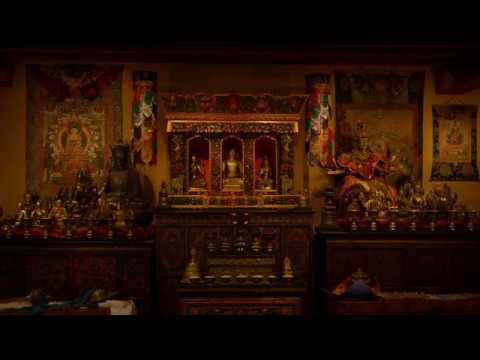In this image of a dimly lit, elaborate interior of what appears to be an old cathedral or church, the room is imbued with a sense of antiquity and reverence. The walls are adorned with ornate artwork and tapestries, potentially depicting portraits of deities, emperors, or celestial beings. On either side of the hall, smaller figurines are mounted, possibly representing relics or sacred symbols. At the center of the room stands a grand altar, intricately decorated with flowers and a prominent gold statue of a deity, reflecting the solemn and sacred atmosphere. Flanking the altar are large, cylindrical columns adorned with various colors, and above them, set within three window-like niches, are exquisitely detailed baby statues. Beneath the altar, in the foreground, are brown wooden benches arranged in neat rows, indicating a space for congregation. These elements together create a deeply spiritual and historically rich environment, characterized by meticulous craftsmanship and reverence for the divine.